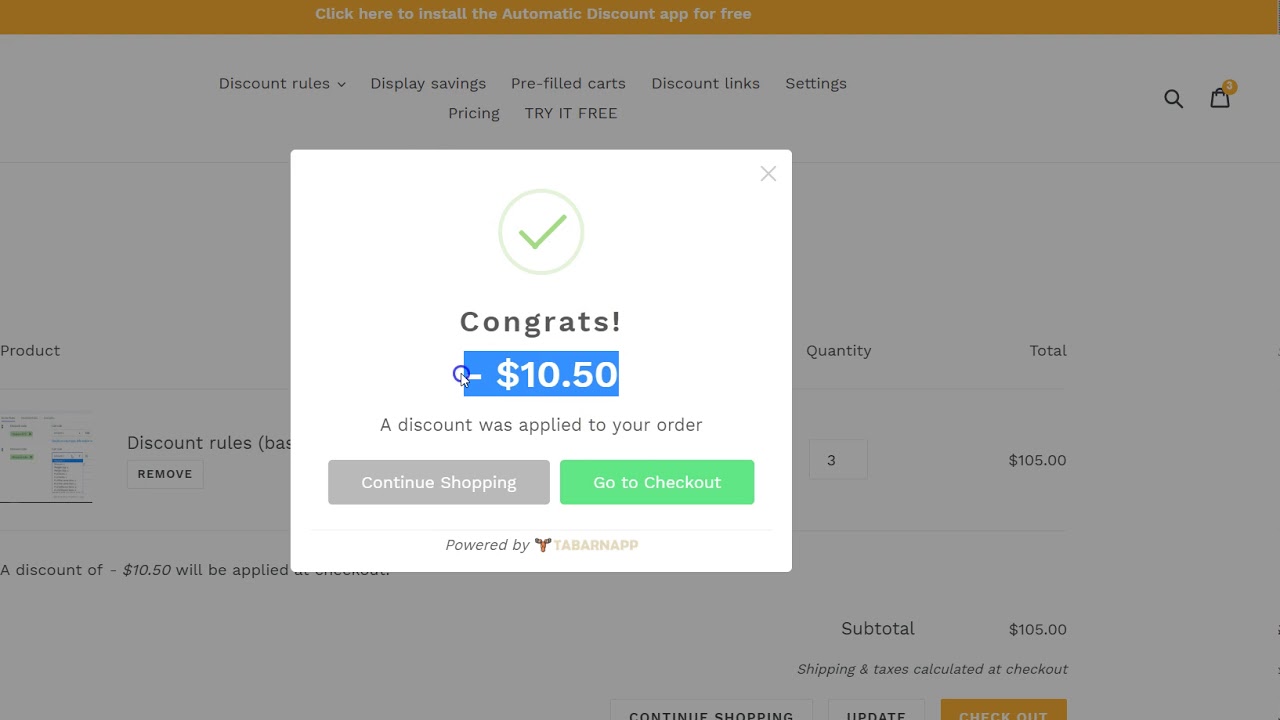Here's a cleaned-up and detailed caption for the described image:

---

A screenshot of a phone screen displays a pop-up notification in the center. The notification features a green check mark enclosed within a gray circle, indicating a successful action. The text within the pop-up reads "Congrats" followed by a message "A discount of $10.50 was applied to your order." Below the message, two buttons are visible: "Continue Shopping" on the left and "Go to Checkout" in green on the right. The pop-up is branded with "Powered by Tab" accompanied by a moose head logo. The background of the webpage features a yellow banner at the top, urging users to "Click here to install the automatic discount app for free." Directly beneath this banner are options in black text for "Discount Rules," "Display Savings," "Pre-filled Carts," "Discount Links," "Settings," and "Try for Free." In the upper right corner of the screen, there is a shopping bag icon with the number 3 inside it, signifying items in the cart, adjacent to a search bar. The main screen displays three active discount rules, collectively totaling $105 in discounts.